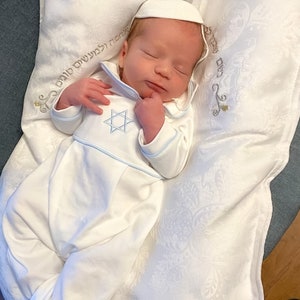The square photo captures a sleeping infant, dressed in all white with a blue Star of David on his chest. The baby, likely a male, is lying on a rectangular pillow adorned with gold embroidery that includes Hebrew text arching around his head and four floral patterns. He is also wearing a small yarmulke. The pillow rests on a greenish-gray rug, which is placed on a wooden floor. The photo's composition has the baby's feet positioned at the bottom and his head at the top of the frame, with his hands gently placed on his chest.